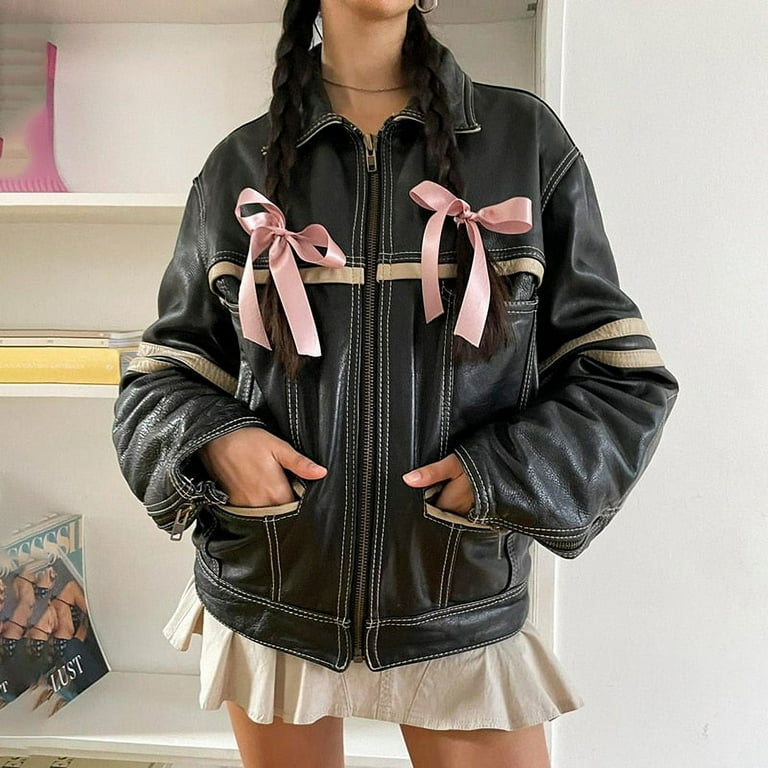This close-up photograph showcases a person's outfit, capturing them from the chin to mid-thigh. The individual's dark hair is styled in two braids, each adorned with a large pink bow resting near the breast area. They are dressed in an oversized black leather jacket, detailed with white stitching that outlines the zipper and the pockets. Beige stripes accentuate the jacket, encircling the elbows and stretching across the upper chest. The person has their hands tucked into the jacket's pockets.

Beneath the jacket, a very short tan skirt is visible. A thin, fine chain necklace, possibly silver or gold, adorns their neck, and a hoop earring can be spotted on their left ear. The background features a white wall on the right and a shelf unit on the left. The shelves hold various items, including papers or books, a pinkish-white vase on the top shelf, a thick yellow book, and a magazine with the word "Lust" prominently displayed on the bottom shelf. This composition suggests a stylish and edgy look, possibly part of a fashion ad.